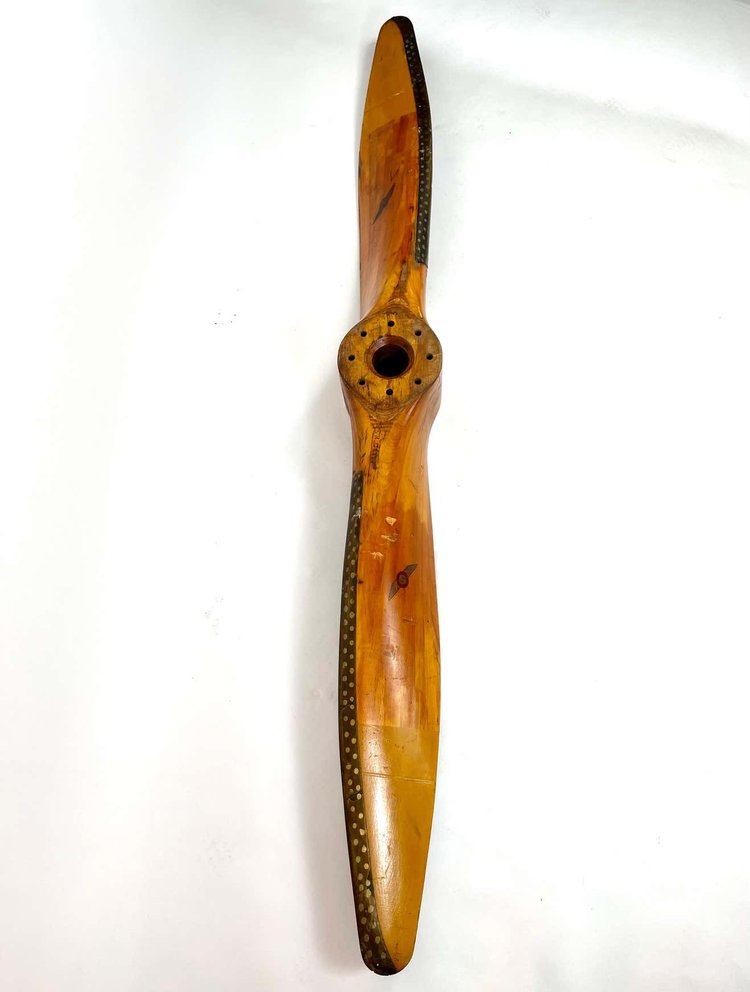This photograph showcases a polished wooden propeller, likely designed for an airplane. The propeller is elegantly positioned vertically against a white background, with its tips aligned at the top and bottom of the image, and the central hub located in the middle. The central circular hub features a large central hole surrounded by eight smaller drilled holes, indicating where it would attach to a mechanized hub. The propeller's blades exhibit a distinctive tapering design, with chamfered edges and a mixture of darker and lighter wood tones. The leading edges of the blades have dark strips, potentially made of hardened wood or reinforced with metal pieces that are drilled and inset. The trailing edges are lighter in color, emphasizing the intricate details of its craftsmanship. The polished finish highlights the smooth curvature of the blades, providing a clear view of the grain and texture of the wood. Light reflections on the lower part of the propeller add a subtle gleam, enhancing the overall visual appeal of this meticulously crafted object.